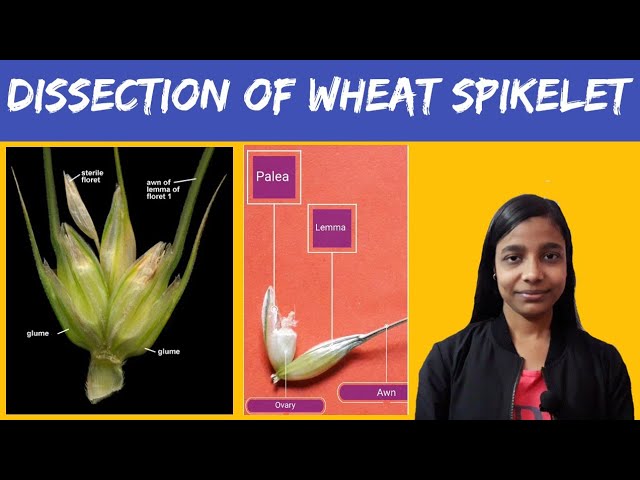This landscape-oriented image features a detailed scientific presentation titled "Dissection of Wheat Spikelet," written in white text on a blue horizontal banner at the top. Below the banner are three distinct panels. The first panel showcases a high-resolution photograph of a wheat spikelet with meticulously labeled parts, including "sterile floret," "lemma of floret one," and "glume," each pointed out by arrows. The second panel presents another close-up of a wheat spikelet section, labeled with terms like "ovary," "lemma," and "palea," set against a peach background. The third panel features a photographic portrait of a young Indian girl with dark hair and brown skin, smiling while looking directly at the viewer. She is dressed in a black jacket and posed against a gold background. The overall design merges realism with graphic design elements.